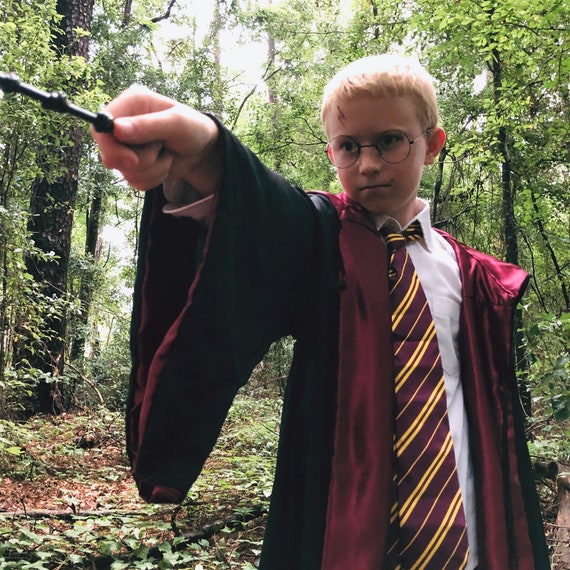The photograph captures a young blonde-haired boy, about 10 or 11 years old, cosplaying as Harry Potter while standing amid a dense forest with tall, thin trees. Dressed in the iconic Gryffindor robes, which are deep black with crimson red pockets and lining, the boy embodies the youthful wizard with meticulous attention to detail. Underneath the robe, he wears a white dress shirt paired with a wide tie in Gryffindor colors—deep crimson with gold stripes. His circular glasses and the painted lightning-bolt scar on his forehead complete the Harry Potter look. The boy is holding the Elder Wand, characterized by its distinctive knots along its length, and he stands with a determined, serious expression on his face. The forest background, dotted with fallen leaves and branches, with glimpses of blue sky peeking through the canopy, adds a magical and adventurous aura to the scene.